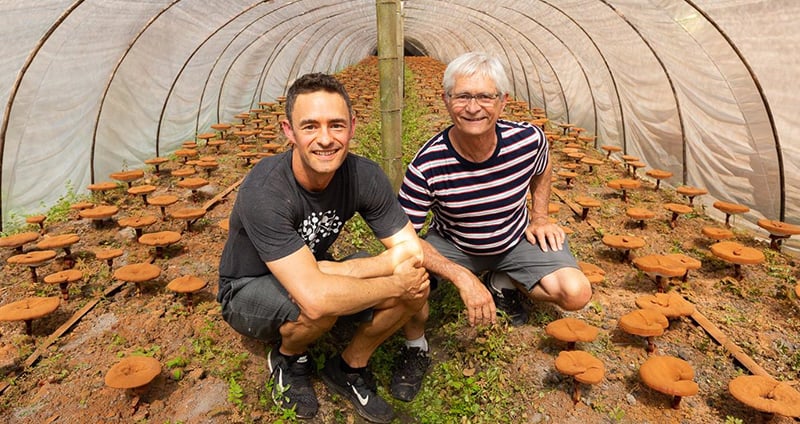In the center of this greenhouse photo, two men are smiling at the camera as they crouch near the ground. The younger man, dressed in a black t-shirt, black shorts, and black Nike shoes, has his arms wrapped around his knee. Beside him, the older man, with short white hair and glasses, wears a black and white striped t-shirt and gray shorts. The greenhouse, characterized by its oval-like tunnel structure made of white cloth material supported by black poles and additional support in the center, stretches far into the background. Surrounding the men and extending throughout the greenhouse are clusters of orange-brown mushrooms, with occasional green grass sprigs visible on the dirt-covered ground.